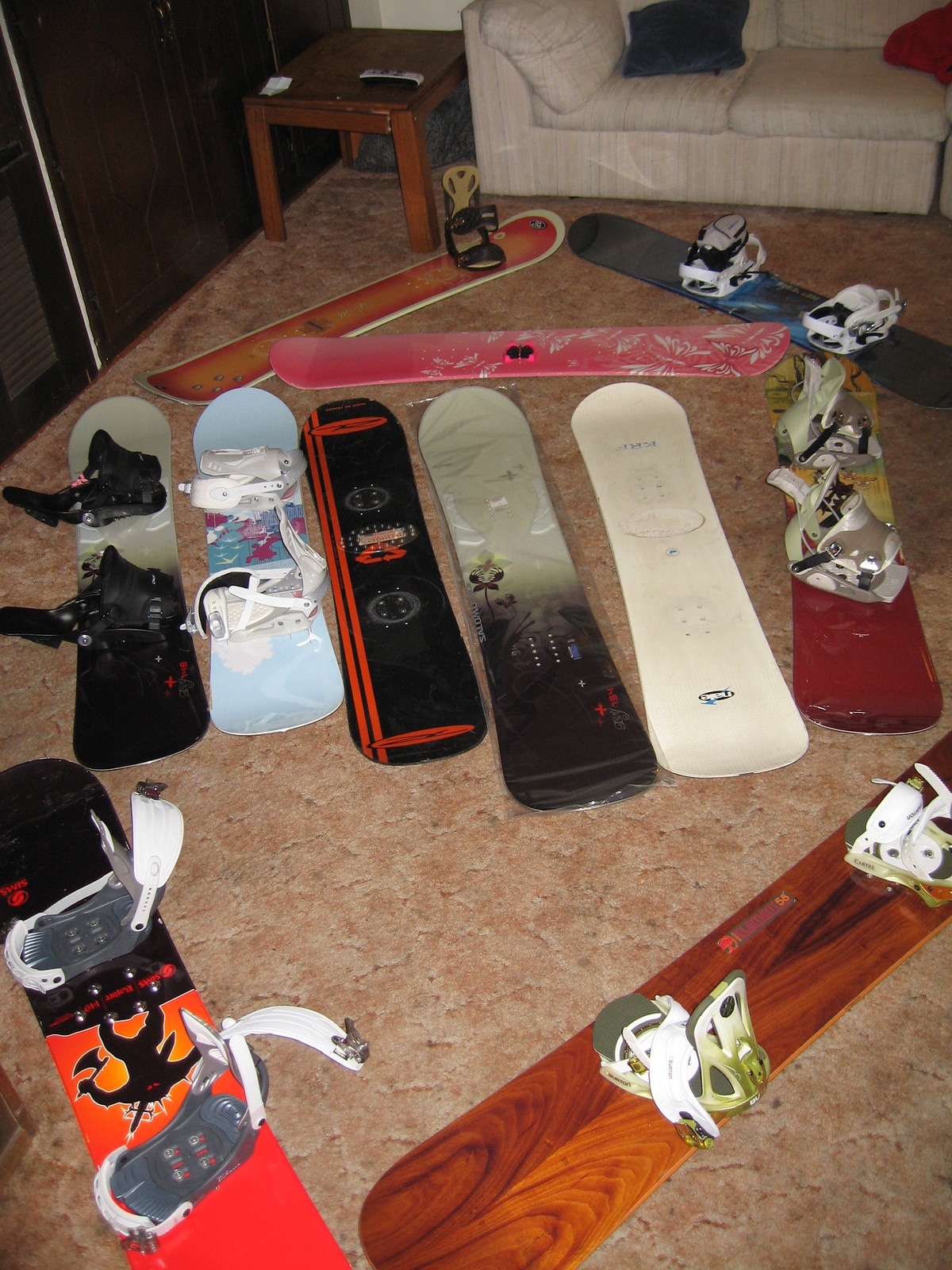In a cozy living room setting, a meticulously arranged collection of eleven snowboards dominates the light brown-beige, sculpted carpet floor. Positioned closer to the viewer are two boards, one diagonal with a wooden finish complete with a foot strap, and another oriented vertically, displaying a striking red-to-black gradient with a ninja figure in the center. In the middle row, six boards are aligned side-by-side. The sequence starts with a green and black board, followed by a light blue one, a black board with orange vertical stripes, a light green and black board, a plain white one, and finally, a vibrant red, yellow, and green board. Of these middle boards, only the first two on the left and the last one on the right have foot straps. Behind this row are three more boards: a pink one lying horizontally, and two meeting at a point to form a V-shape—one is orange and red with a single foot strap, and the other is blue and black with white accents. In the background, an off-white couch adorned with blue and red pillows (or perhaps a red blanket) sits next to a simple wooden side table holding a remote and a piece of paper. The setting is completed with a dark brown closet door with vents against a black wall.